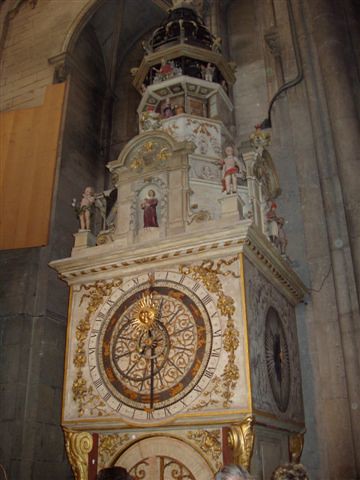Inside the majestic cathedral stands a large, ornate clock, a striking masterpiece of craftsmanship. The cathedral's interior is adorned with intricately carved gray granite stone walls that exude a timeless elegance. The clock itself is a stunning blend of artistry and opulence, featuring beautifully carved wood that has been meticulously painted white and lavishly gilded in gold and red. 

The top of the clock is a breathtaking tableau, adorned with depictions of various saints and cherubs that ascend in a staggered fashion, creating a visually captivating ascent that culminates in a grand dome. The clock's face is encircled by a band of gold gilding, enhancing its regal appearance. Surrounding the face is elegant trim in shades of gold and brown, adding to the clock's rich detailing.

The numbers on the clock face are uniquely represented as intricate swirls, contributing to the overall ornate design. The clock hands are a striking combination of gold and black, standing out prominently against the white face. Flanking the main clock, additional elements are visible, suggesting the presence of a calendar, artfully integrated in a round format. This exquisite clock is not only a functional timepiece but also a magnificent piece of art that enriches the splendor of the cathedral.